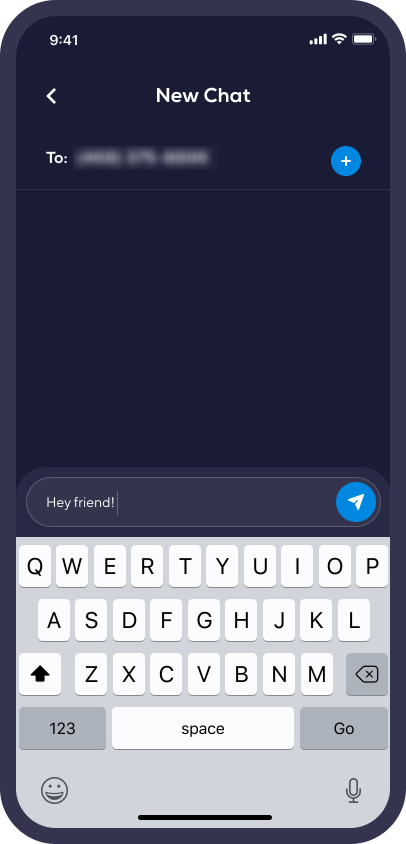This digital image showcases a smartphone screen with the time displayed at 9:41 at the top. In the upper right corner, there are icons indicating a Wi-Fi connection and the battery level. The screen shows a messaging app, with a left arrow button labeled "New Chat" and a blurred-out name accompanied by the number "2". A prominent blue and white plus button is visible on the interface. A text message has been typed, reading "Hey friend!" followed by an exclamation point. To the right of the text input field, there's a blue and white send button featuring an arrow. The on-screen digital keyboard is also visible, displaying the QWERTY layout: the top row with the letters Q, W, E, R, T, Y, U, I, O, P; the middle row with A, S, D, F, G, H, J, K, L; and the bottom row with Z, X, C, V, B, N, M.